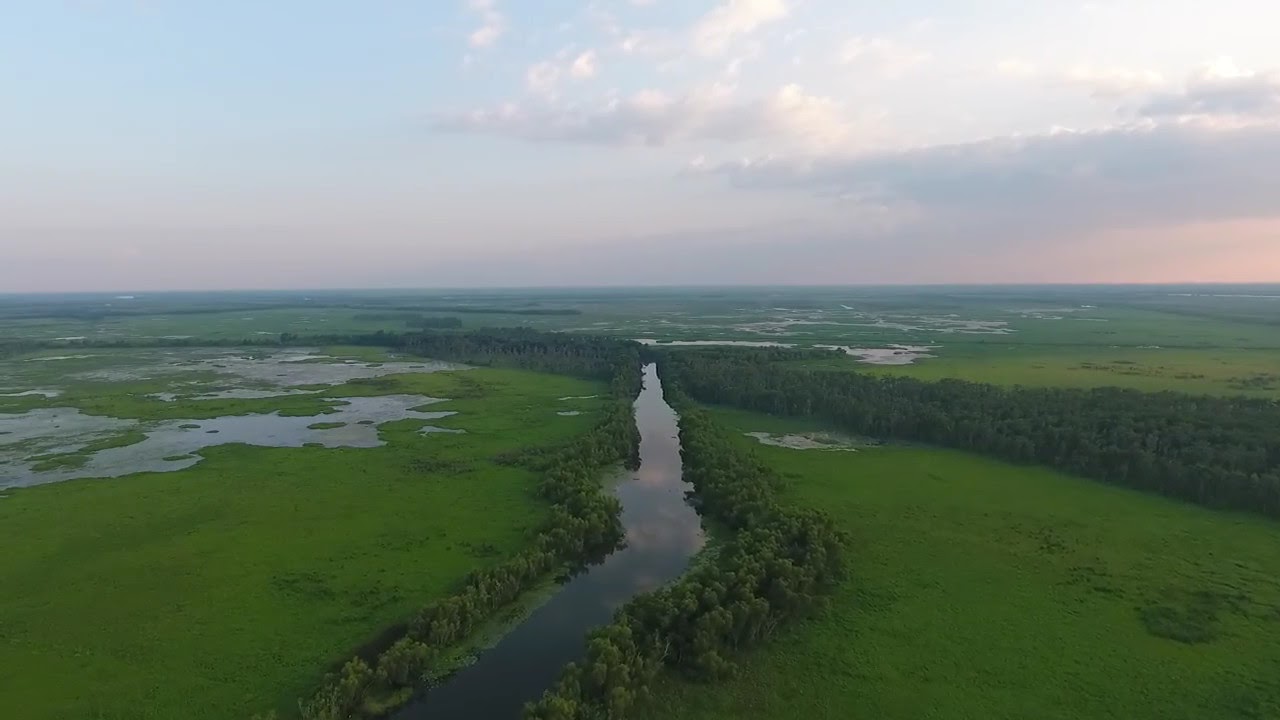This aerial photograph captures a sprawling, flat landscape dominated by a sinuous river that weaves from the bottom left through the center before snaking off into the distance. On either side of the river, vast stretches of grassy wetlands and sloughs can be seen, with shallow patches of water interspersed throughout. The river is framed by dense clusters of trees that line its banks, forming extensive wooded areas. The sky above is a vibrant tapestry, with the left side featuring a blue hue that transitions to a violet-pink color toward the upper right, suggestive of a sunset. The scene exudes a serene, natural beauty well-captured from a high elevation.